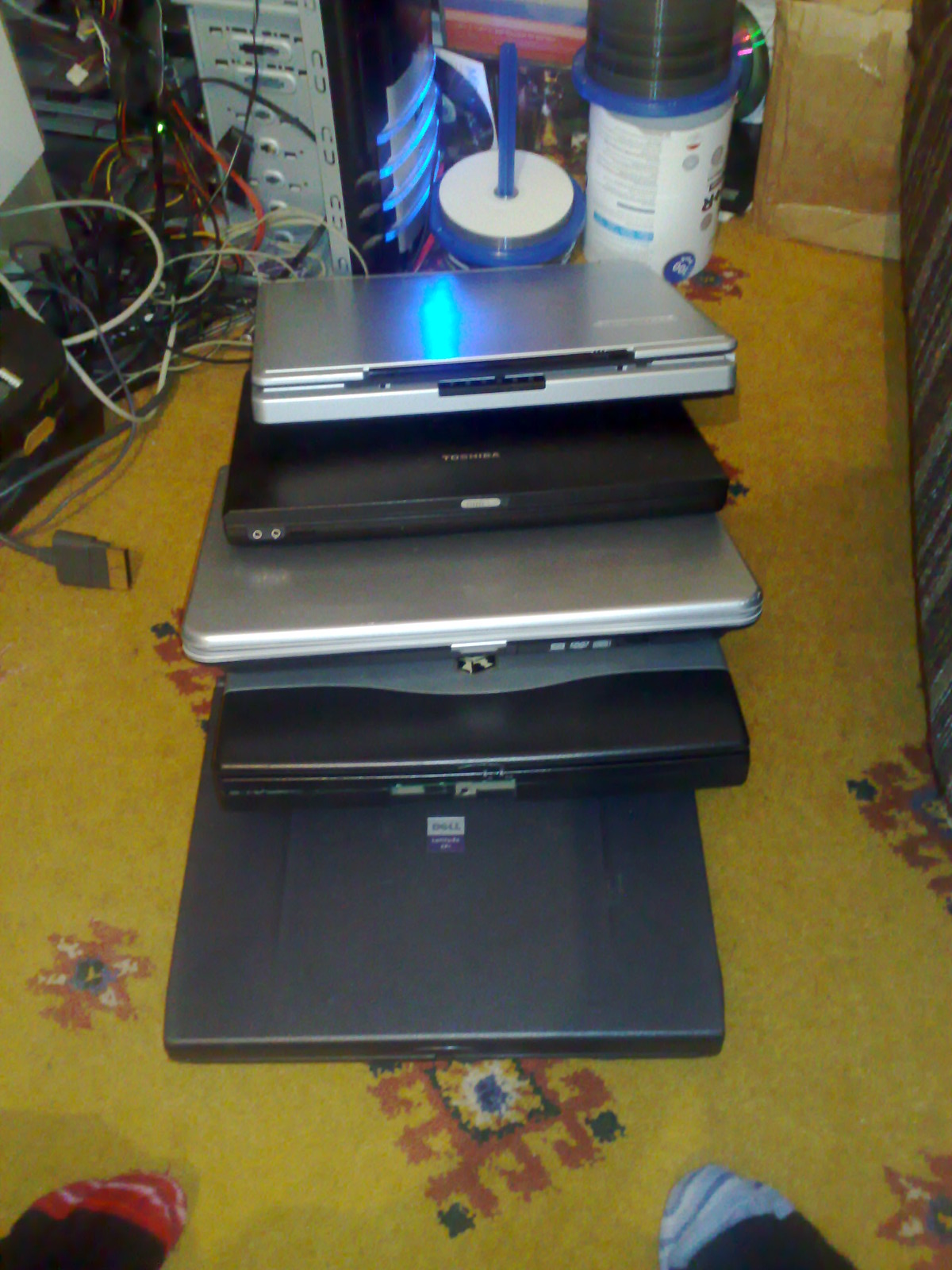The image displays a detailed scene of assorted computer equipment atop a mustard yellow carpet, which features a periodic reddish and black patterned design. Prominently in the foreground, there is a stack of five electronic devices, likely closed laptops, varying in color—silver, black, silver, black, and gray. Among them, one Toshiba laptop stands out, identifiable by its visible headphone and microphone jacks. Also visible are brand names like Dell. Beside these devices, partially fanned out, are several electrical cords, predominantly white with one bright red cord catching attention, and a blue spindle holding numerous CD-ROM disks. Furthermore, another tall stack of CDs rests on a white cylinder. The background reveals a large, open-chassis desktop computer with loose wires spilling out and decorative neon blue bars on its front, reminiscent of a high-end gaming system. Adding a human element, the image captures the tips of a person's sock-clad feet at the bottom—one sock with a blue tip, the other with a red tip—suggesting the photographer's presence in the scene.